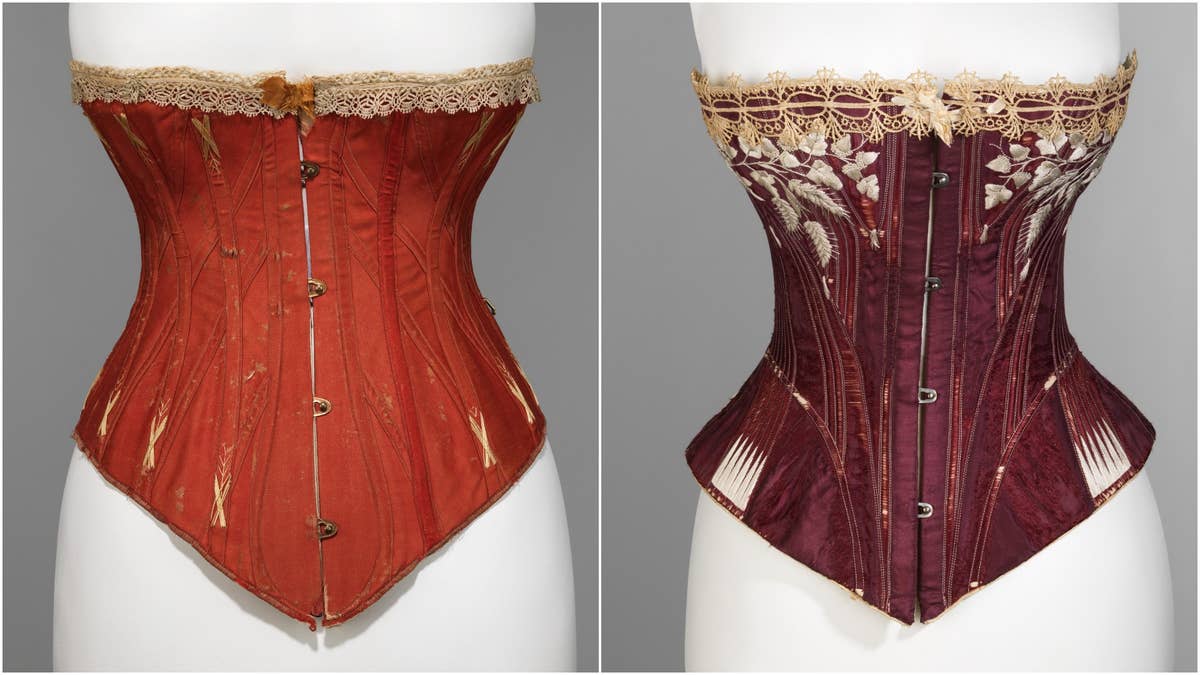The image features two side-by-side photos showcasing corsets on headless white mannequins, cropped just above the shoulders and at the thighs. Both corsets are tightly fitted with four button-like fasteners down the front. The left corset is a striking burnt orange or reddish-brown color, adorned with a gold bow and white lace at the top. It also has brown ruffles just beneath the bust, adding a touch of elegance. The right corset is a rich burgundy or deep purple, featuring intricate white leaf and grass-like patterns along its sides. It is similarly designed with beige lace trimming the top and brown ruffles. Both mannequins stand against a neutral gray background, highlighting the detailed textures and colors of the corsets.